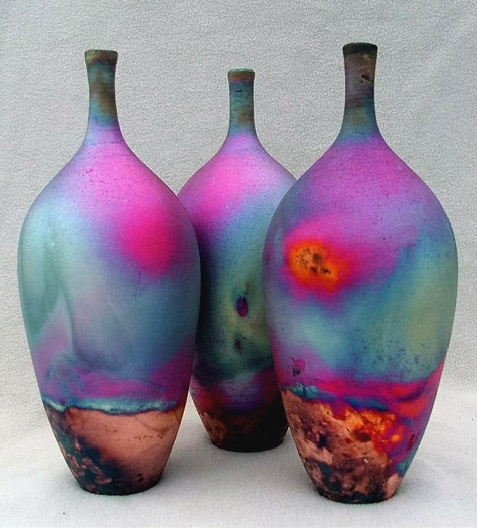This full-color, vertically rectangular photograph captures a staged indoor scene under artificial lighting. The background features a textured gray wall and a white countertop with no noticeable border. In the foreground, three vividly colored vases—possibly glass or ceramic—are arranged, their striking design immediately drawing attention. These vases resemble bowling pins with their narrow, short necks and wide shoulders tapering off towards the base, evoking the shape of water jugs or even wine bottles. Each vase boasts a mesmerizing, almost psychedelic blend of colors: the lips and necks are adorned with darker hues, while the bodies display a tie-dye-like pattern predominantly featuring shades of blue, red, and purple. The lower sections blend into a marbled mix of brown, red, and orange tones. Together, these vases create a harmonious and visually captivating set, resting on the countertop without any text or figures in the scene.